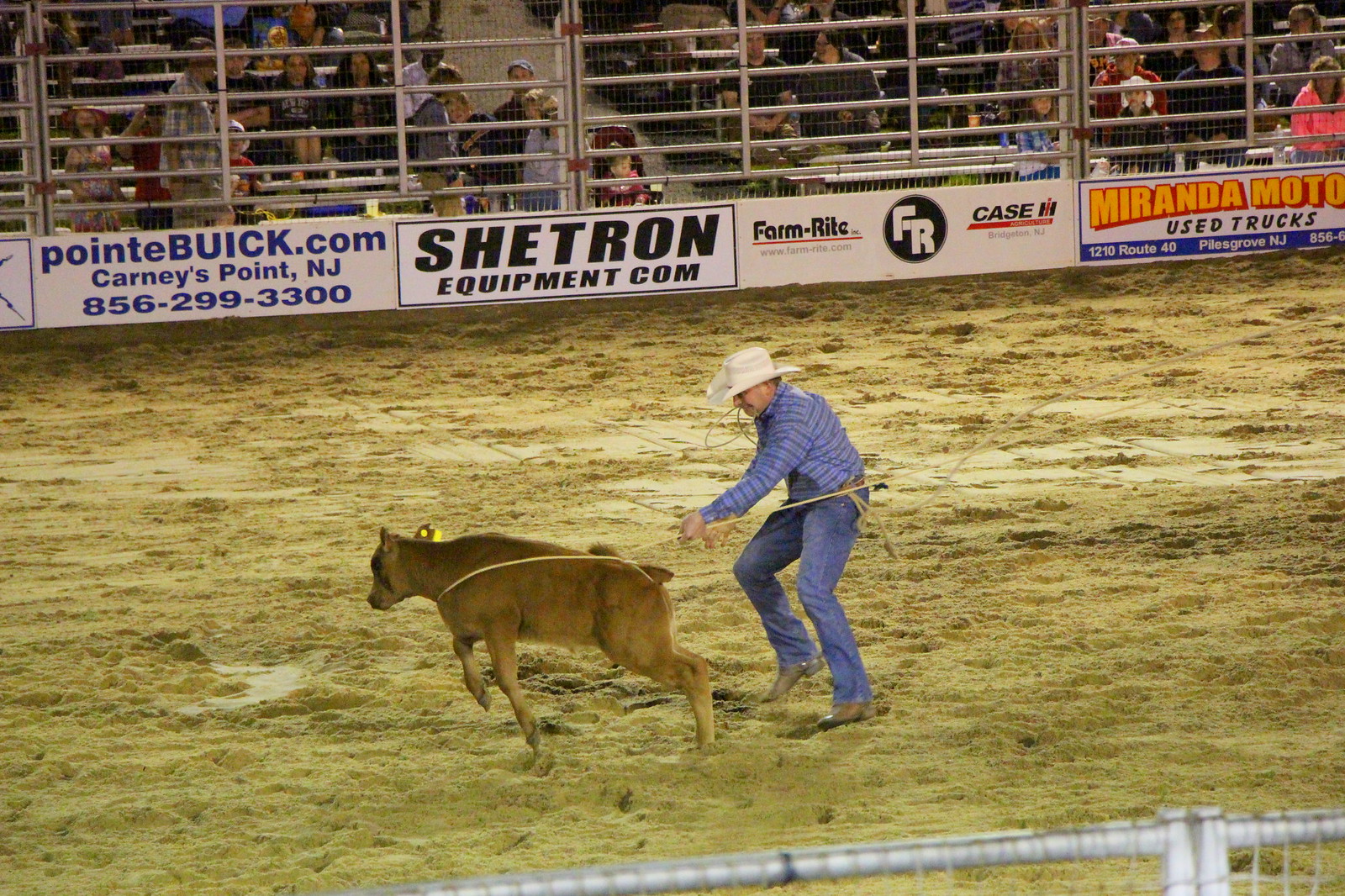In the center of this dramatic rodeo scene, a cowboy dressed in a white cowboy hat, a blue plaid shirt, blue jeans, and classic cowboy boots skillfully ropes a young brown heifer. The rope is securely fastened around the heifer's neck, lifting its feet into the air as the cowboy pulls it towards him in a display of traditional rodeo prowess. The action unfolds on a dirt arena, surrounded by metal fencing. In the background, numerous spectators eagerly watch from behind the upper right fence, contributing to the lively atmosphere. Along the lower and sides of the fence, various advertisements can be seen, including those for pointbuick.com, chatronequipment.com, Farm Right, and Miranda Motors' used trucks in bold yellow lettering on a red background. The scene is a vivid representation of the rugged and competitive spirit of rodeo culture.